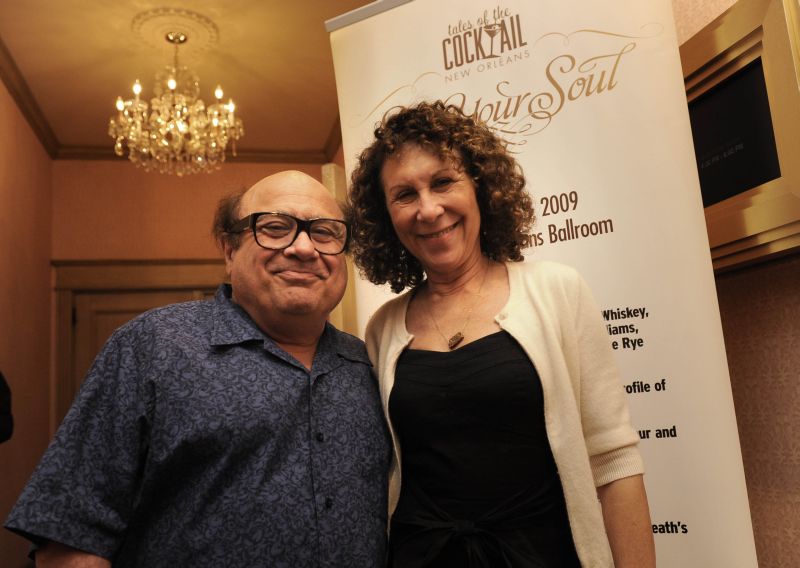In the image, a celebrity couple, Danny DeVito and Rhea Perlman, are standing and smiling directly at the camera, positioned centrally. The setting appears to be an indoor cocktail party in New Orleans, specifically the event "Tales of the Cocktail" held in 2009. Just behind them, slightly to the right, is a clear sign reading "Tales of the Cocktail, New Orleans, Your Soul, 2009, Ballroom." Overhead in the top left of the image, a fancy, illuminated chandelier casts a warm glow, and beneath it, a door is visible. Danny DeVito is dressed in a dark shirt with a black pattern, while Rhea Perlman wears a black dress paired with a white sweater. The room has a beige-colored wall with an empty picture frame on the right. The overall color palette of the scene includes blue, black, white, gold, silver, tan, and brown.